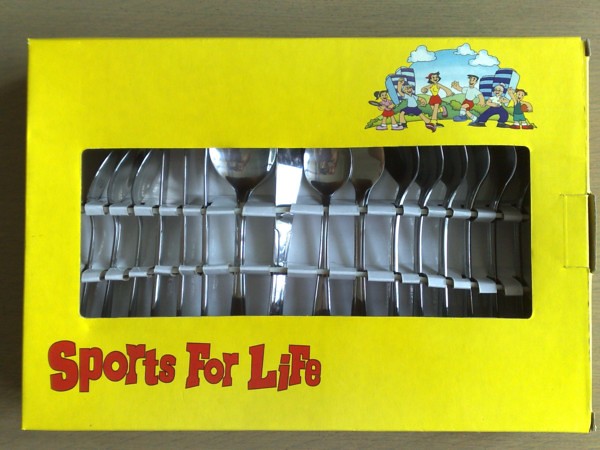The image is a color photograph of a bright, neon-yellow cardboard box, set against a nondescript khaki, green, or brown-gray background. The box prominently features the red block text "Sports for Life" in the bottom left corner. In the center of the box is a rectangular opening that reveals a set of silverware, including several spoons and a central knife, held securely in place by a slotted strip. The handles of the silverware are arranged in two rows on a white slab. The upper right corner of the box contains a cartoon-style illustration depicting people outdoors. In the illustration, under a blue sky with scattered clouds, several individuals are shown walking or running on green grass. Some of these figures are wearing track shorts and t-shirts; notably, a woman in a yellow tank top and red shorts, and a man in a white t-shirt and red shorts. Blue flags with light and dark blue stripes are also visible in the background of the illustration. The scene appears to be illuminated by direct light shining from above, particularly highlighting the central knife.